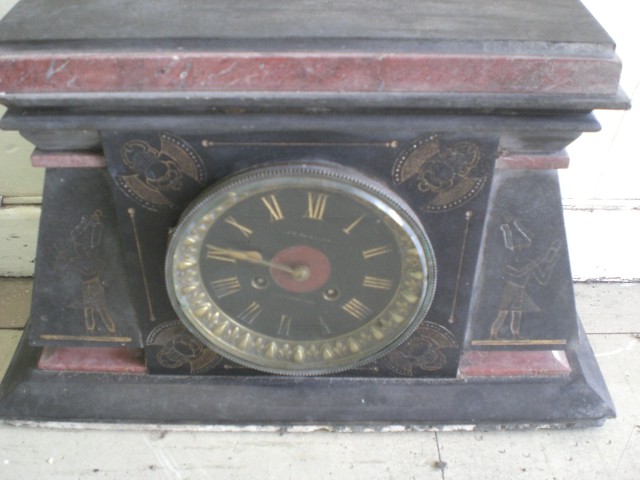A meticulously designed square-shaped clock is prominently featured in this image. The central circular clock is encased within a striking black and red square frame, creating a bold visual contrast. Flanking the clock on both sides are pieces of artwork, though they are blurred and indistinct. The clock sits atop a light gray platform, further enhancing its prominence. The clock's face is adorned with elegant golden Roman numerals and matching golden hands, which add a touch of opulence and classic sophistication to the overall design.